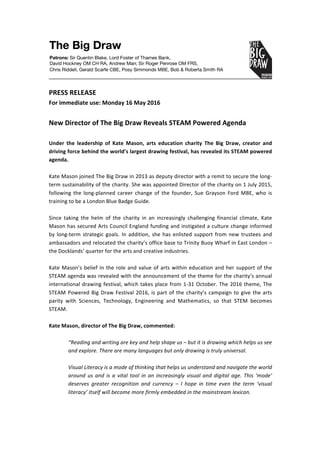The image is a front-facing screenshot of a black-and-white press release dated Monday, 16th May 2016, from the arts education charity, The Big Draw. The press release, titled "New Director of The Big Draw Reveals STEAM-powered Agenda," introduces Kate Mason, the new director. Under Mason's leadership, The Big Draw, known for creating and driving the world's largest festival, has adopted a STEAM-focused agenda. Additional text on the page includes detailed paragraphs about Mason's vision and plans, along with her comments on the new initiatives. The document appears in black text on a white background, emphasizing key details about the leadership transition and future directions.